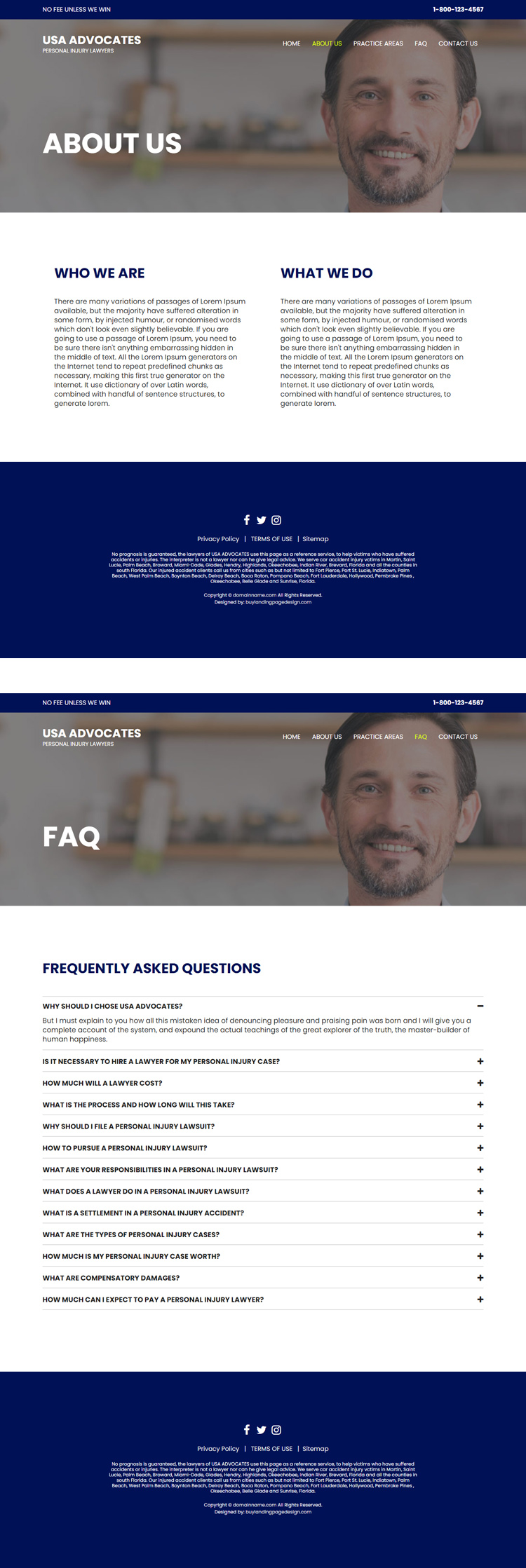This image appears to be a screenshot of a website depicting two similar sections, one above the other. Each section starts with a narrow dark blue border at the top, containing text on both the left and right sides, which are unfortunately unreadable due to their small size. Below the blue border is a semi-translucent grayish area. 

On the left side of this gray section, the text "USA Advocates" is visible, and directly below that, in larger letters, is "About Us." Adjacent to this text is a blurred image of a man's face set against a background that includes a wall with wooden shelves filled with indistinguishable items. 

Beneath this is a white area featuring two columns of text. The left column is titled "Who We Are," and the right column is titled "What We Do," though the detailed contents of these paragraphs are unreadable.

At the bottom of each section, there is a large rectangular area in navy blue, populated with an array of white text. This section includes identifiable symbols for Facebook and the platform formerly known as Twitter, among other unreadable text. 

Below this first section is a repeated structure, beginning with the same image of the man and a heading that reads "Frequently Asked Questions." Below this heading are a series of clickable questions intended to help users with various issues, though the specific questions themselves are not legible. The section concludes with the same navy blue rectangular area as the first.